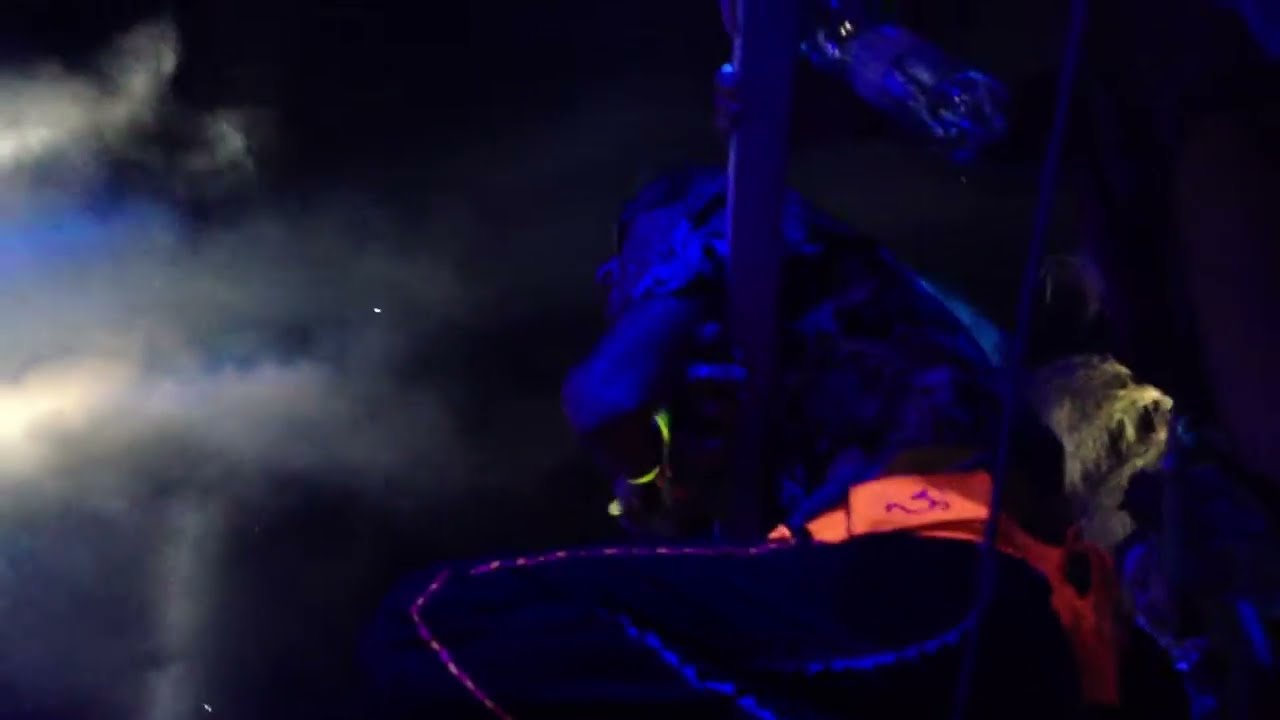The image is extremely dark and challenging to decipher, suggesting it might be a screenshot from a video game. The background is predominantly black, making the details difficult to discern. On the left side, there is some gray smoke or clouds set against a purple background. In the center, an ambiguous deep blue silhouette is visible, vaguely resembling a creature or structure, but its indistinct form leaves much to interpretation. Just below the center, a red or faded red belt with a symbol resembling a "U" with a hook is visible, possibly indicating attire.

On the right of the image, a green mass can be seen, adding to the scene’s complexity. Also on the right, it seems we are looking up at someone, perhaps a person with glasses, wearing a short-sleeve shirt and an orange strap in the belt area. This individual appears to be leaning over a bar or railing, with an arm extended over it, suggesting a perspective from below. In the upper part, another hand is visible, possibly holding a soda bottle, contributing to the sense of proximity and interaction.

Towards the bottom of the image, there is a curved blue line, vaguely reminiscent of a road or another form, and an outline that could be interpreted as part of a leg, again adding to the image’s enigmatic quality. Overall, the dark, blurred, and smoky environment makes it incredibly difficult to pinpoint specific features with certainty.